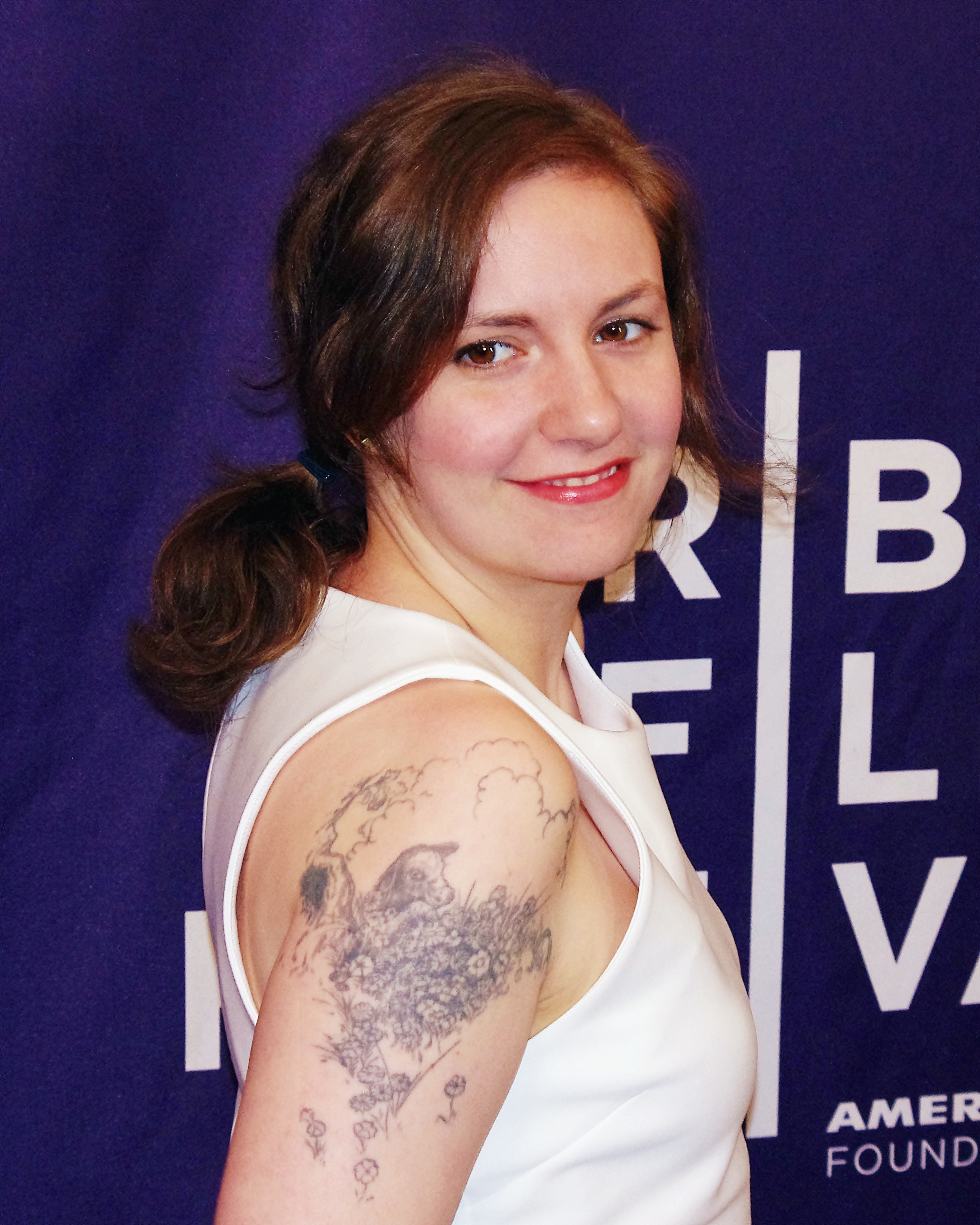The photograph captures a young woman in her early twenties with brown hair pulled into a side ponytail that includes a black braid. Her face, highlighted by pinkish-red lipstick, faces forward with brown eyes glancing directly at the camera, while her body is angled to the right. She wears a sleeveless white blouse, and her right arm, the only one visible, features a black outline tattoo depicting a sheep in a field of flowers. The background consists of a dark blue fabric banner adorned with multiple lines of white text, though most of the writing is obscured by her figure. Partial letters visible include R, B, F, L, V, A, M, E, R, F, O, U, N, T. She exudes a gentle smile, adding a touch of warmth to the image.